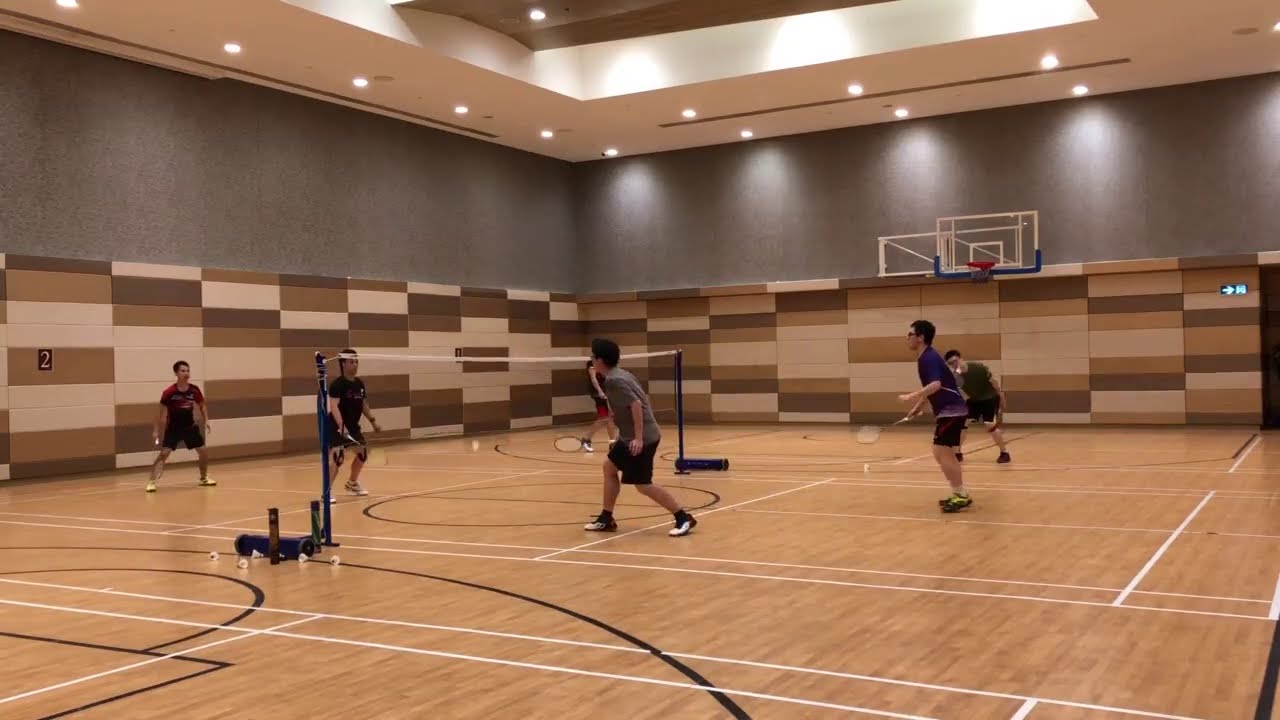In this digital photograph, four men are playing badminton in a multipurpose gymnasium. The standard light tan floor, marked with white lines, indicates it can also be used for basketball, and a hoop is visible in the background. The center of the court features a badminton net. To the right, two of the male players wear gray and blue shirts respectively, while on the left, the other two sport darker shirts. The gym's upper walls are solid gray, while the lower part displays a checkered pattern of white, light brown, and dark brown rectangles. Numerous small but bright lights illuminate the scene from the ceiling, and birdies are scattered across the floor, indicating an active game. An exit sign and additional basketball equipment also feature in the background.